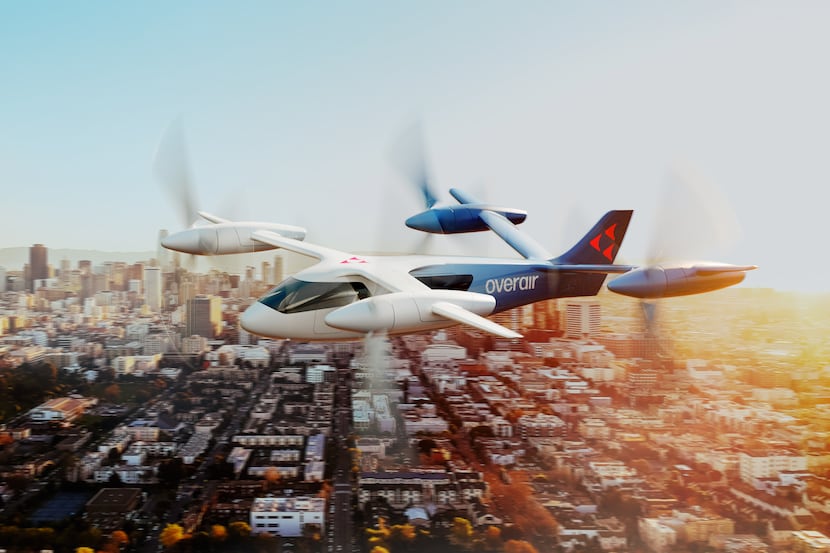This image captures a futuristic, computer-driven drone with a design reminiscent of both a plane and a helicopter. The drone, flying towards the left side of the frame, is blue and white in color with a white text reading "over air" and a distinctive red triangle logo on its tail. It features four wings, each equipped with propellers. The drone appears to have windows and a sheer window in the front, offering a modern and advanced aesthetic.

Below the drone lies a sprawling cityscape, characterized by a mix of tall and shorter buildings, roadways, and patches of greenery. The buildings are predominantly gray and white, and the city seems well-developed, possibly modern or slightly futuristic. In the far background, a small mountain range can be discerned under a light blue sky, emphasizing the drone's elevated flying altitude.

The overall scene combines elements of modern urban living with advanced aerial technology, all set under a clear, blue sky.